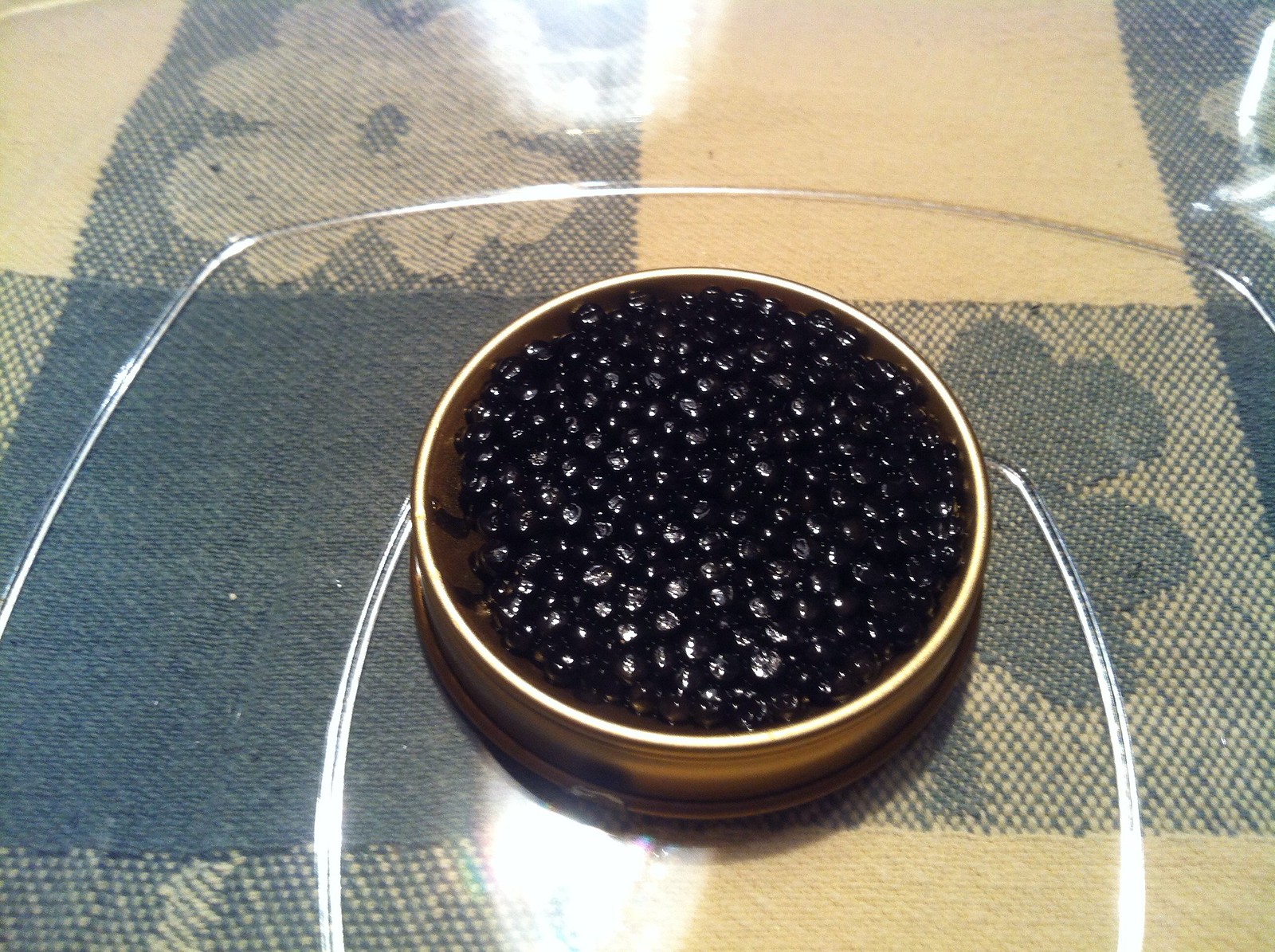This photograph showcases a meticulously arranged setup featuring a circular metal dish, likely containing black caviar, placed atop a large, translucent glass plate. The dish itself is a light gold color with a shiny gold rim, adding a luxurious touch to the presentation. The caviar, comprised of small, glossy black eggs, glistens under ample lighting, suggesting a well-lit scene that's reflected in both the caviar and the glass plate. The plate rests on a distinct fabric tablecloth that features a quilted or checkered pattern, alternating between white and various shades of blue, and adorned with flowers in some of the squares. The overall image emphasizes the contrast between the dark, shiny caviar and the light, patterned background, with reflections adding depth to the composition. No utensils or additional elements are visible, keeping the focus squarely on the elegant display of the caviar dish.